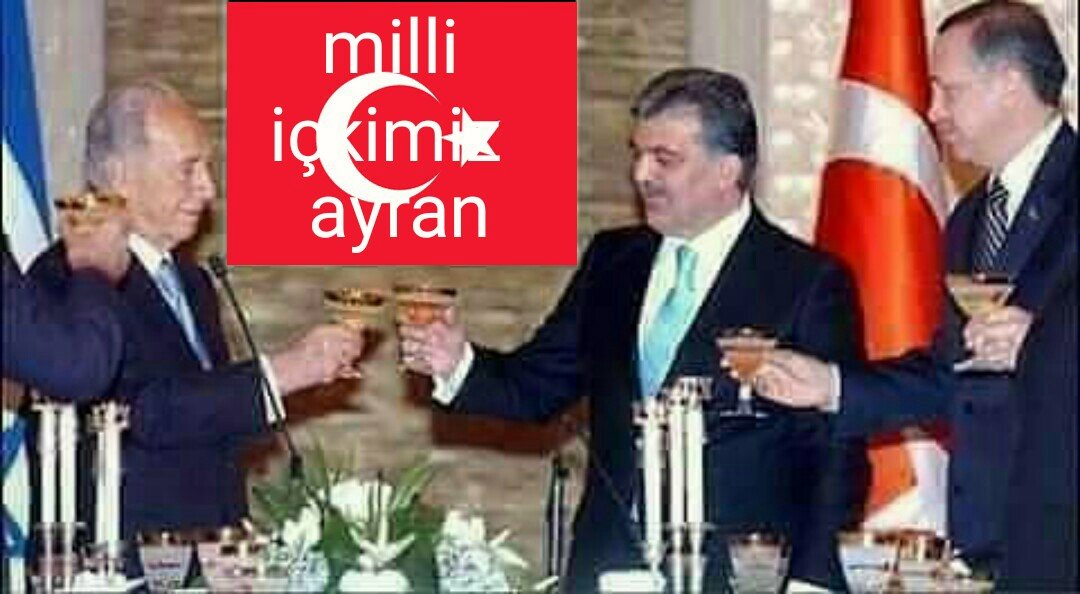This color photograph, taken in landscape orientation, captures a formal gathering of three men at a dining table, each raising a glass of champagne in a toast. The men, who appear to be of European descent, are all dressed in dark suits with white collared shirts and ties: the man on the left in a blue suit with a blue tie, the man in the center in a black suit with a light blue tie, and the man on the right in a black suit with a black and white checked tie. The table in front of them is adorned with crystal glassware, candles, and flowers, adding a touch of elegance to the scene. Behind them, to the right, is a red and white flag, and to the left, a blue and white flag. In the center background is a red square with white text in Turkish, featuring a crescent moon and star emblem. The overall style of the image is photographic realism, depicting a moment of camaraderie among these likely political leaders.